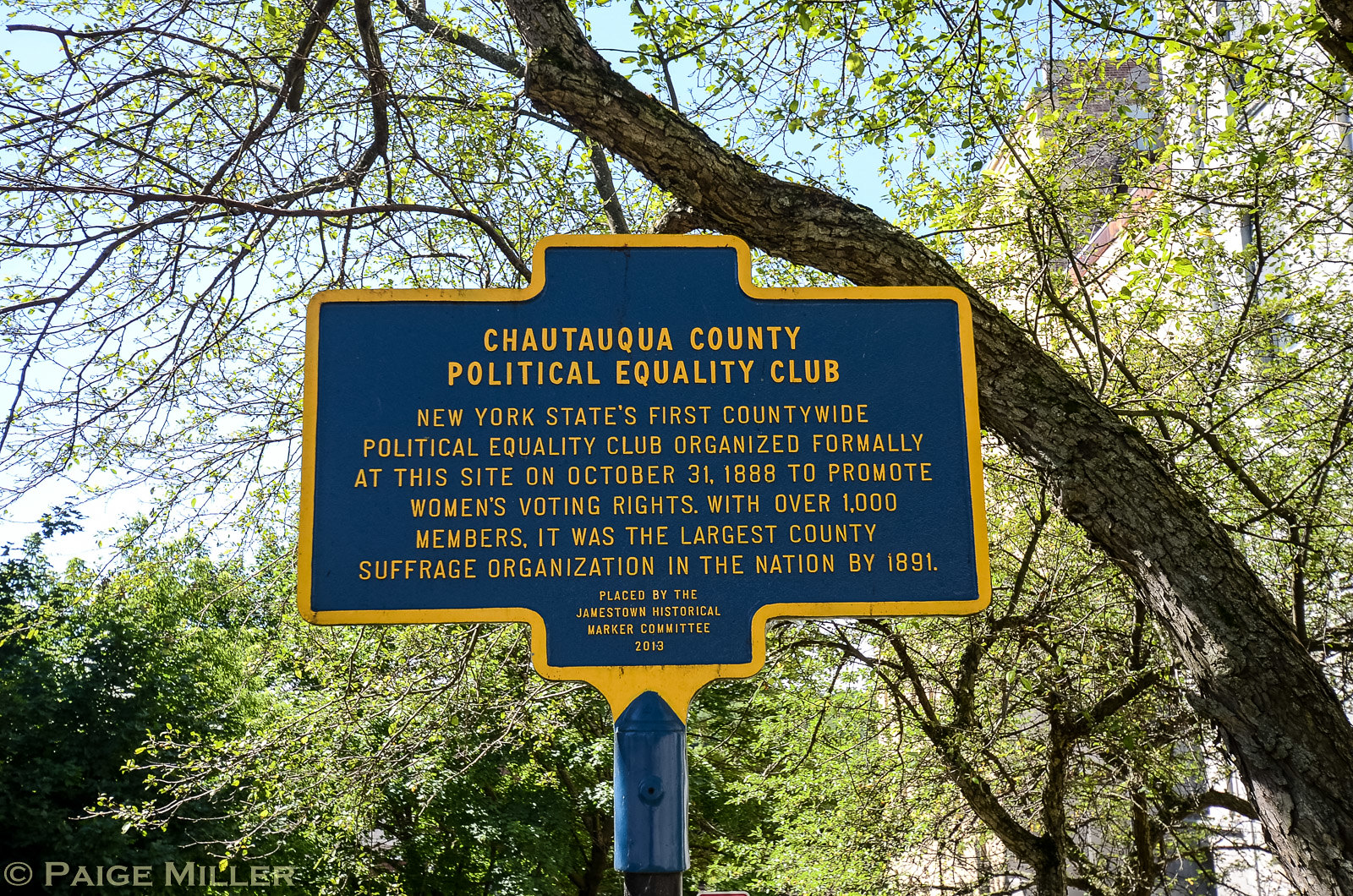The image captures an outdoor scene dominated by a prominent blue and yellow historical marker in the center. The metal sign, featuring a blue background with a yellow border and text, commemorates the Chautauqua County Political Equality Club, New York State’s first countywide political equality club, formally organized at this site on October 31, 1888, to promote women's voting rights. With over 1,000 members, it grew to be the largest county suffrage organization in the nation by 1891. The marker was placed by the Jamestown Historical Marker Committee in 2013. In the background, the right side of the image features urban elements, including tall, barely visible apartment buildings obscured by a layer of branches and sparse green leaves. A large tree extends diagonally from the bottom right to the top left, with various branches and tiny budding leaves. Additional foliage and bushes are visible in the lower left corner. The photograph also includes a small watermark at the bottom left, indicating © Paige Miller.